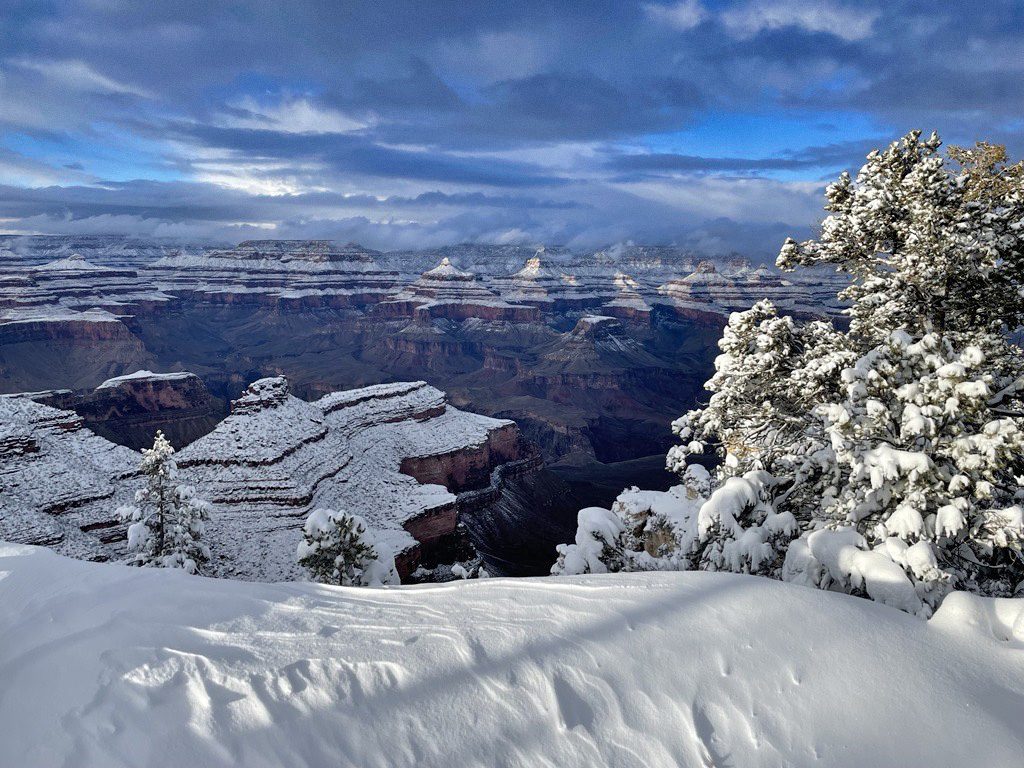This photograph captures a breathtaking wintertime scene at Bryce National Park. In the foreground, the viewer stands atop a snowy peak, gazing out into the iconic canyons and striated stone mountains of the park. Dominating the right side of the picture is a large evergreen tree, its branches heavily laden with snow, with hints of green needles peeking through. To the left, smaller trees sprinkled with snow contribute to the frosted landscape. The center of the image showcases the dark, snow-free canyon depths in contrast to the snow-covered ridges of the surrounding peaks, which resemble culinary confections iced in white. The sky above is covered in dark purplish-gray clouds with occasional patches of light blue peeking through, adding to the wintry atmosphere. The dominant colors of the scene are whites, grays, browns, and green, making for a striking and serene winter tableau.